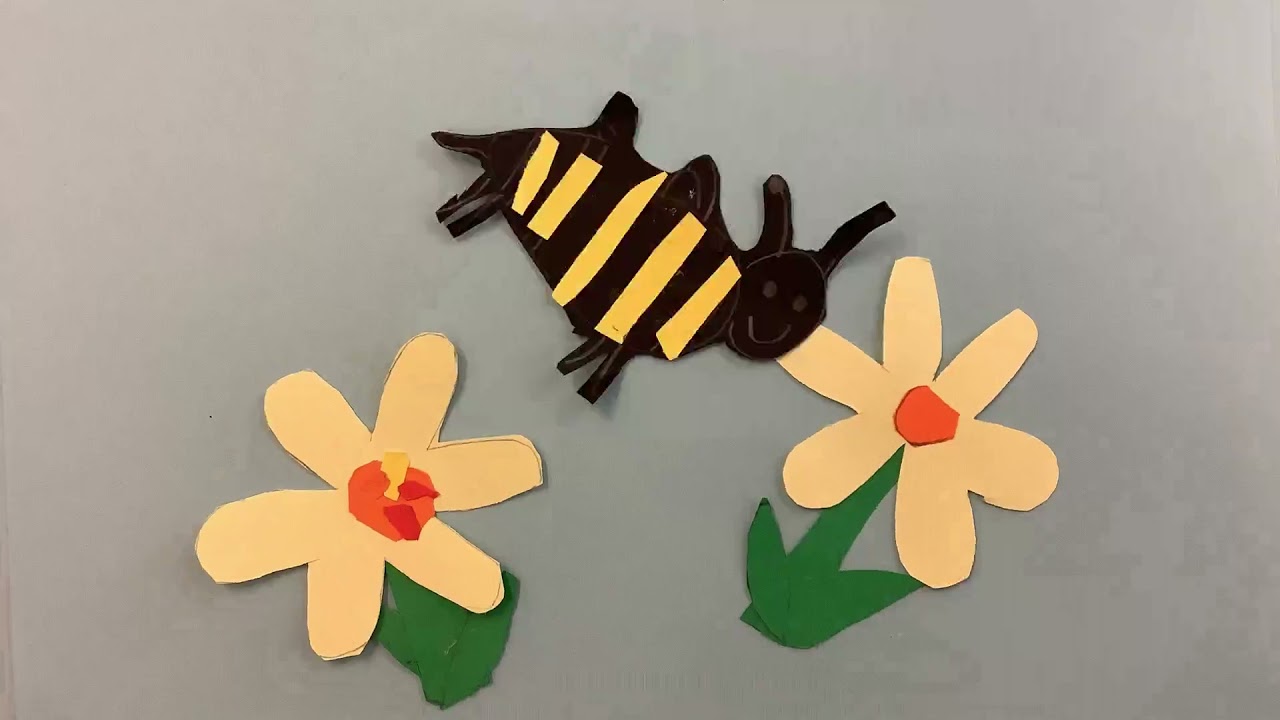The image features a light purple piece of paper adorned with intricate cut-out figures. There are two flowers, each with six petals in a light beige hue. The first flower has a vibrant center that blends shades of red, orange, and yellow, complemented by a green stem and leaves. The second flower showcases a solid orange middle, also supported by a green stem and leaves. Additionally, the composition includes a cut-out of a black animal, distinguished by its yellow stripes along its sides. This animal figure appears to have a couple of humps on its back, a short tail, and notably long ears.